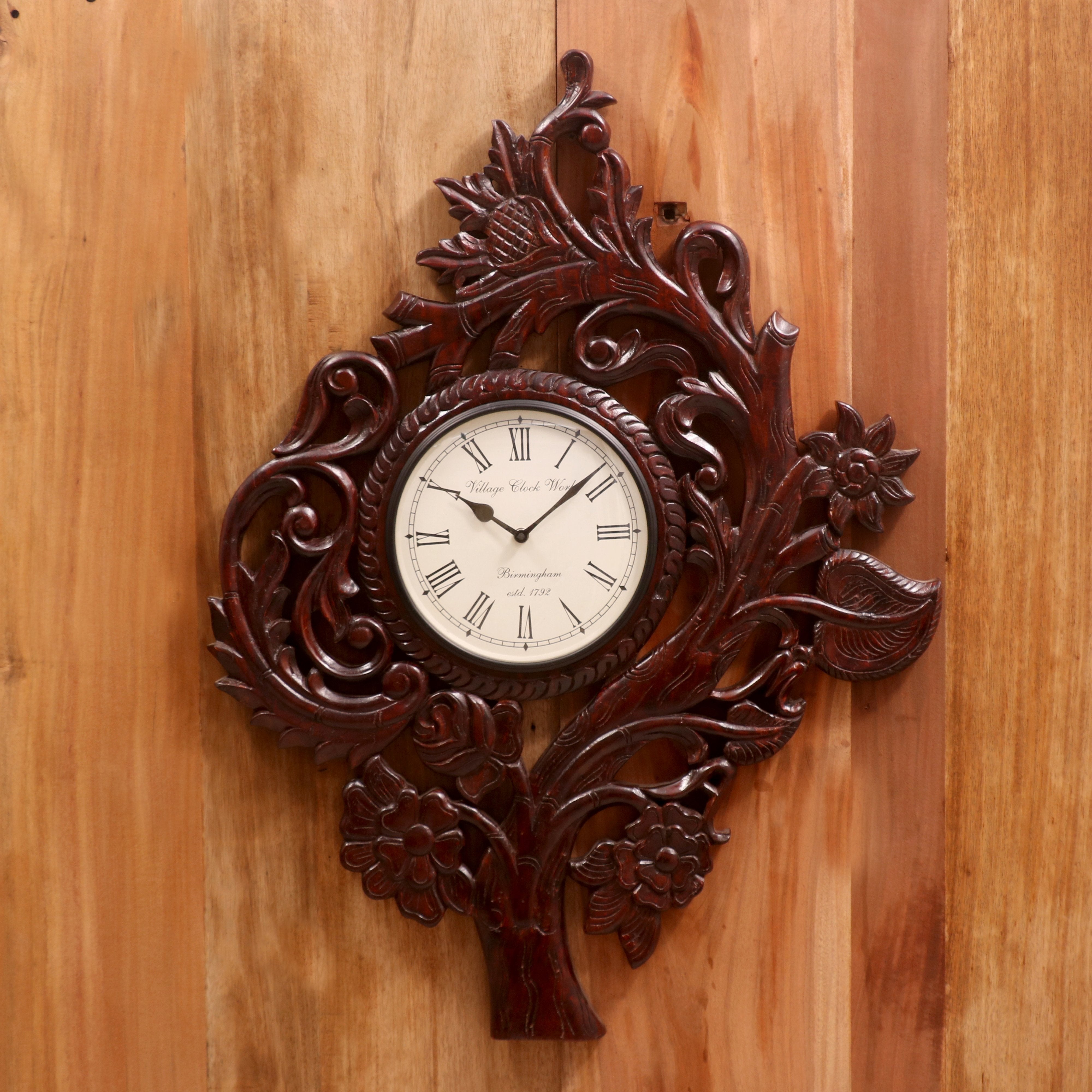This square, photographic image showcases an elaborately carved wooden clock mounted on a vertically planked wooden wall. The wall is made of light brown wood, while the clock itself is crafted from darker wood. The clock face, which is beige with black Roman numerals, indicates a time of approximately eight minutes after ten. Encircling the clock face is an intricate, diamond-shaped carving depicting a tree, complete with branches, leaves, and flowers. At the base of the carving, there is a tree trunk extending downward. The dial of the clock is black, and the face bears the inscription "Village Clock Works, Established 1792" in cursive, with the word following 'Village Clock Works' being somewhat difficult to decipher. The overall design is ornate, with numerous floral and leafy details embellishing the tree motif.